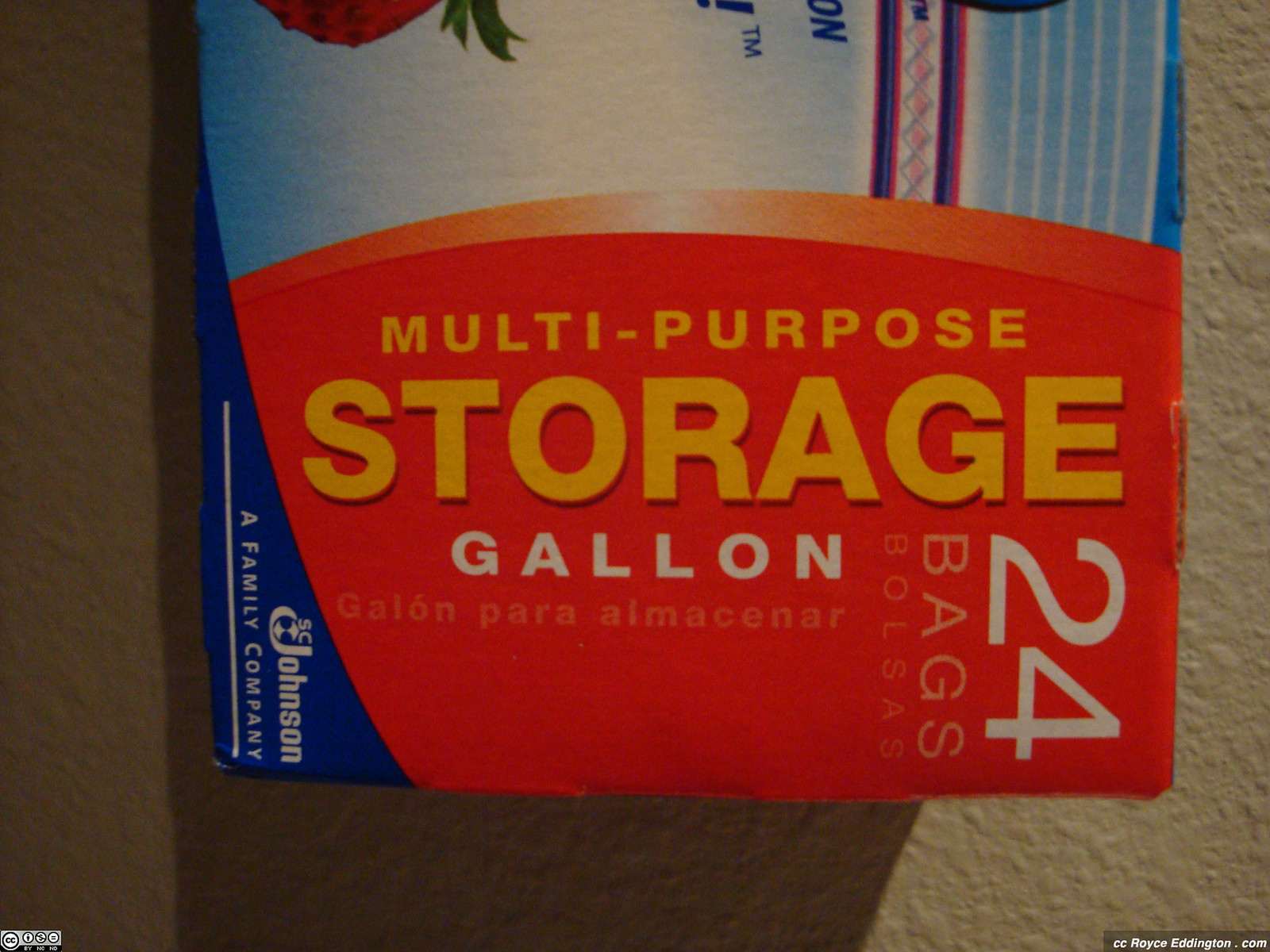In the photograph, there is a package of gallon-size storage bags prominently displayed against a simple background. At the bottom of the image, a white website stamp is visible. The package features a vibrant design with a navy blue, white, and pink color scheme. The bottom section of the package is highlighted in red-orange, with labeling in both white and gold fonts. The text reads "24 bags" in white font, "gallon" also in white, and "multi-purpose storage" in gold. Above this section, a partial view of a strawberry is depicted, adding a fresh, appealing touch to the packaging. Additionally, at the bottom of the package, "SC Johnson, a family company" is written in white font, underscored by a clean white line. The box casts a shadow on the surface it rests on, giving the image a sense of depth and realism.